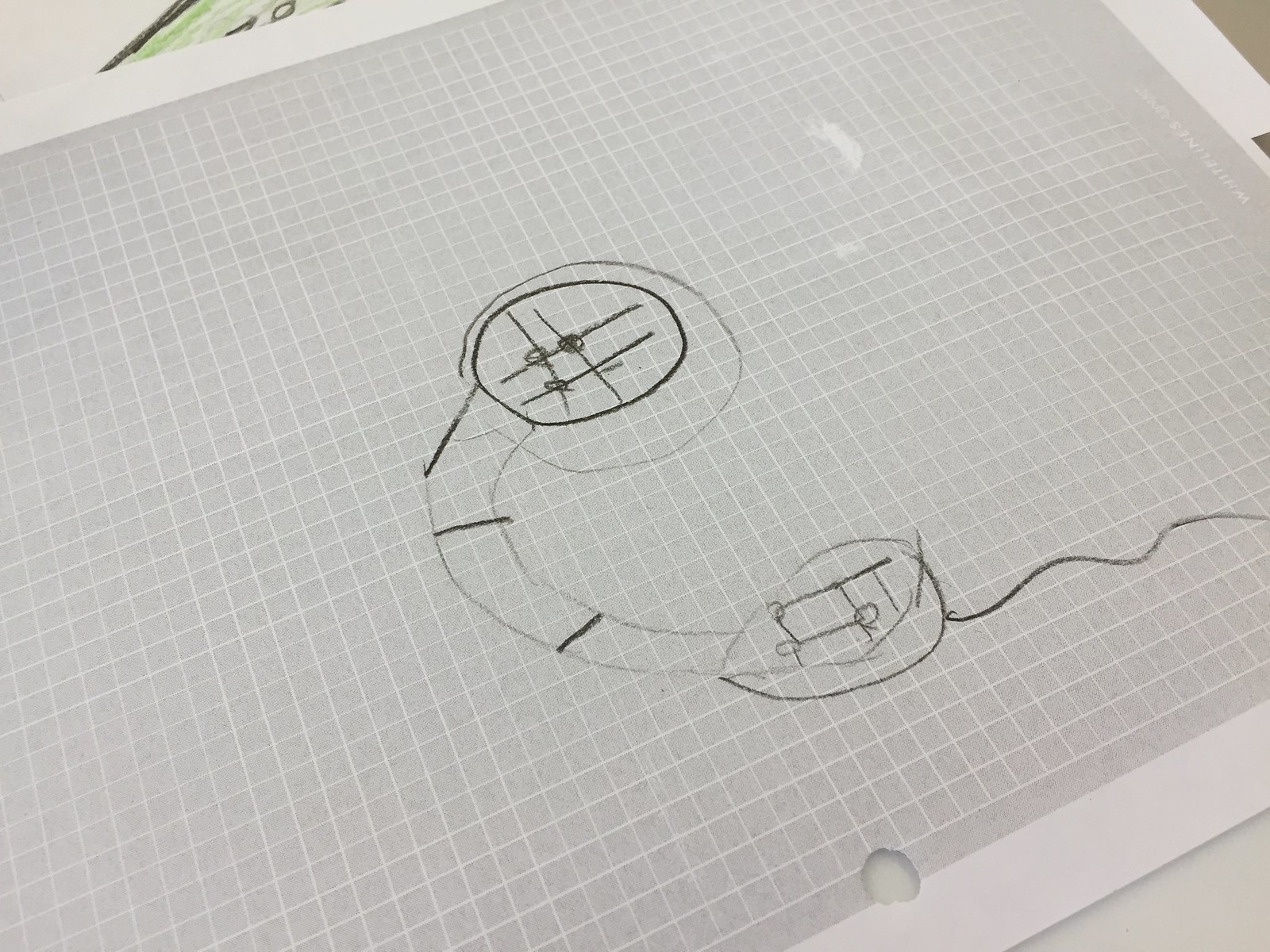The image features a large piece of gray graphing paper with small white grid lines, lying on a white table. The paper has a white outer border giving it a framed appearance. At the center of the graphing paper, a detailed drawing is rendered in black pencil.

The drawing consists of two circular shapes, one positioned above the other, connected by a curved, tube-like structure resembling a slide, which is segmented into three distinct sections by divider lines.

Inside the upper circle, a tic-tac-toe-like grid is drawn with smaller circles occupying the four corners and the center square. The lower circle contains a similar grid, but only three of its corners are occupied by small circles. From the side of this lower circle, a thin, squiggly white line extends outwards.

Additionally, a circular hole is present near the bottom edge of the graphing paper, possibly the result of a hole punch.